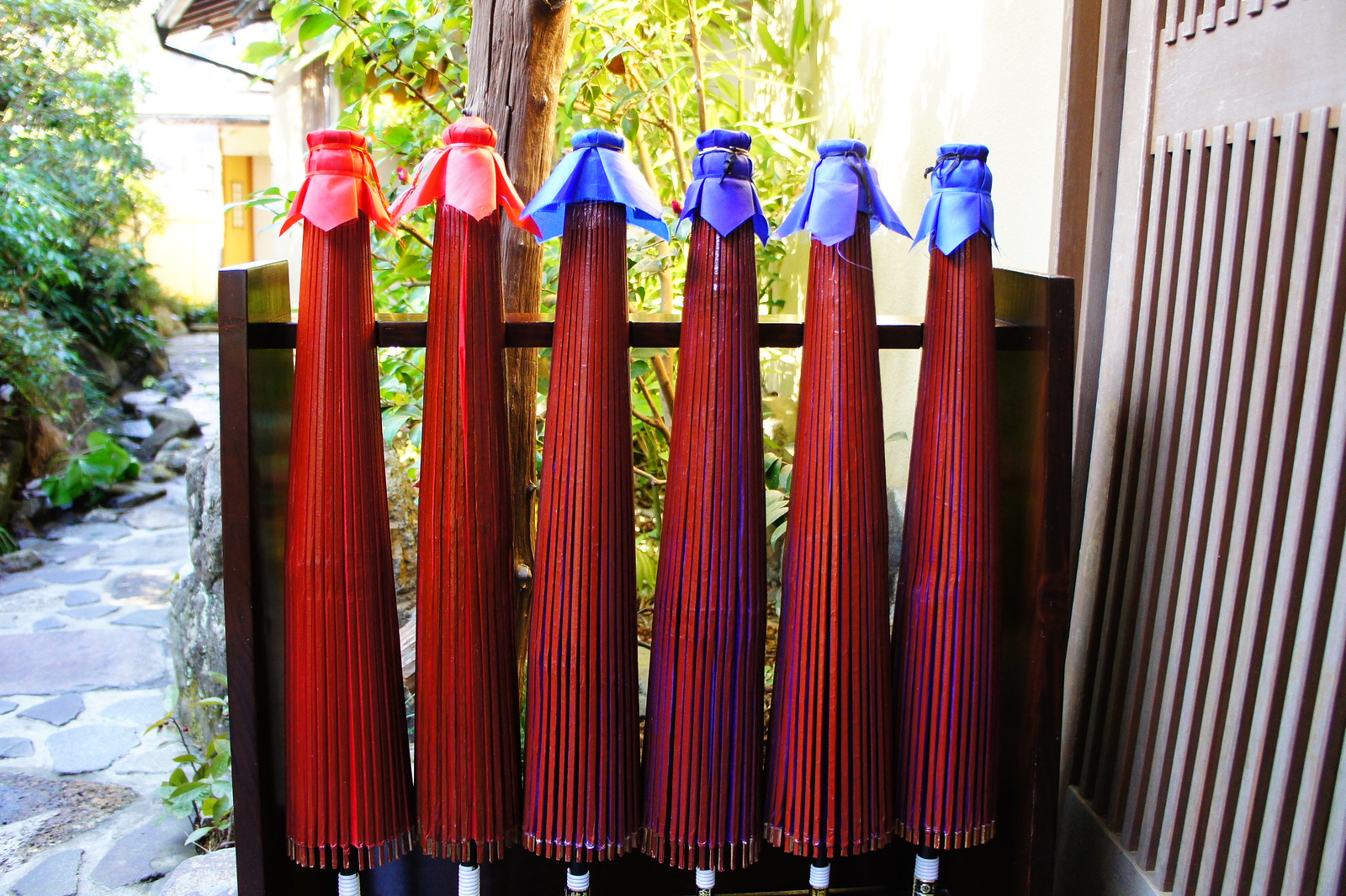This detailed photograph captures a peaceful outdoor scene, focusing on a neat arrangement of six oriental-style umbrellas leaning against a dark wooden rack. These umbrellas are crafted in an unusual design, possibly for ornamental use or as parasols rather than for rain protection. Each umbrella sports a vivid red fabric and prominently features large, visible red spokes. At the tops of the umbrellas, decorative caps made of fabric are tied on—a detail that accents their unique aesthetic. The two umbrellas on the left have red caps, while the remaining four, extending to the right, are capped in a light blue fabric.

The scene is set on some sort of a patio or porch area with a stone path dotted with greenery leading off to the left. To the right of the rack, there's the wall of a house or possibly a restaurant. The setting is serene, nestled within a garden-like environment, with stone slabs and masonry forming the path. Additional components of the background include green and lighter green bushes, giving the scene a refreshing, natural ambiance. This well-arranged image blends elements of sophisticated craftsmanship with the tranquility of an outdoor space.